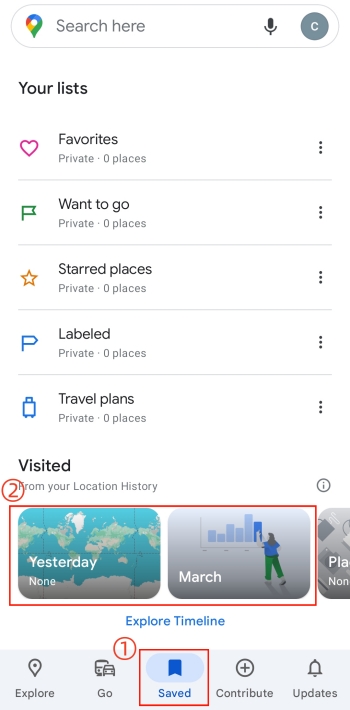This image is a screenshot from a cell phone, featuring the Google interface, and is in portrait orientation without a defined border, mimicking the proportions of a cell phone screen. The background is predominantly white. 

At the top, there is a long horizontal oval search bar with the Google Pinpoint icon, displaying the colors red, blue, green, and yellow. Within the search bar, the text "Search here" is presented in grey on a white background. To the right of this, there are two icons: a microphone icon and a grey circular avatar featuring the letter "C" in white font.

Below the search bar, the heading "Your lists" is written in black. Under this heading, there are several list options, each accompanied by a small icon on the left and text in black on the right, with ellipsis dots to indicate additional options. The lists are arranged as follows:
- A flag icon with the label "Want to go"
- A star icon with the label "Starred places"
- Another flag icon with the label "Labeled"
- A suitcase icon with the label "Travel plans"

Following these categories is the section titled "Visited", which features a box labeled "Yesterday" and another labeled "March" with a red outline, a number "2" inside it, and a small bubble in the upper left corner.

At the very bottom of the frame, there is a grey toolbar with various options. The "Saved" option is highlighted with a blue circle, indicating it is currently selected. This option is also marked with a red rectangular box containing the number "1" in red within a circle, signifying a count or alert associated with this selection.